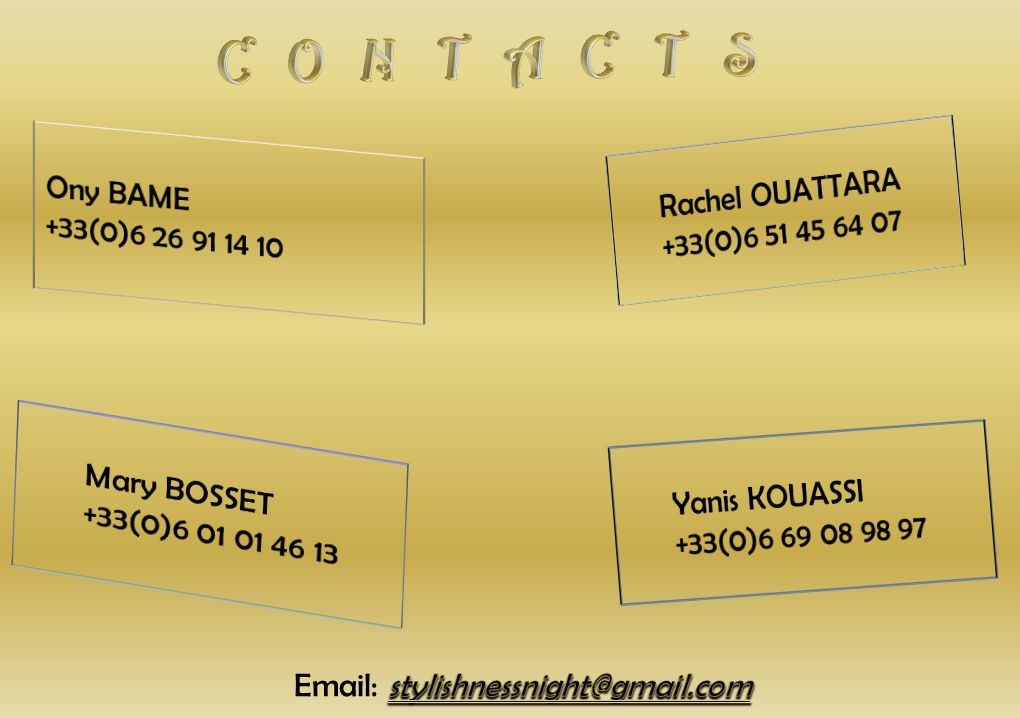The image is a computer-generated, rectangular graphic with a gradient yellow background featuring darker shading throughout. At the top, in ornate gold and white capital font, the word "CONTACTS" is prominently displayed. Each corner of the image contains a sunken, outlined rectangle, each listing a name and a phone number in black text. The top-left rectangle displays the name "ONY BAME" and a corresponding long phone number, suggested to have an Indian format due to its length and "330" extension. The top-right rectangle features "RACHEL OUATTARA" and her phone number. In the bottom-left rectangle, the name "MARY BOSSETT" appears with a phone number underneath. The bottom-right rectangle shows "YANIS KOUASSI" alongside a phone number. The image concludes with the word "EMAIL" at the bottom center, followed by an underlined email address for linking purposes, "stylishnessknight@gmail.com". The rectangles are slightly angled, giving a dynamic layout to the contact information.